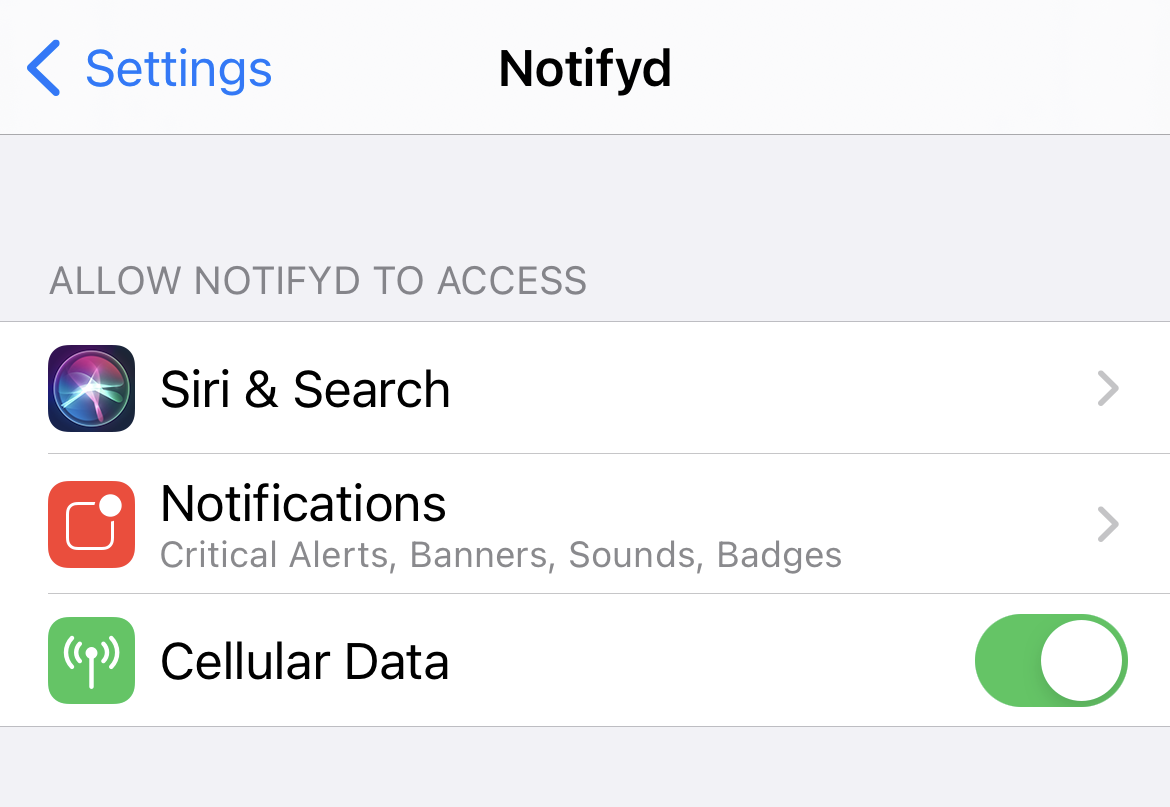This image is a detailed screenshot of the settings menu for an app called "Notyfyd" (spelled N-O-T-I-F-Y-D) on a smartphone. The title "Notyfyd" is prominently displayed at the top of the screen. Below the title, there are multiple options denoted, reflecting the permissions and settings that the app can access. 

The first option listed is "Siri & Search," which has an arrow on the right-hand side, indicating that more options can be accessed by tapping this entry. 

Following that, there is a section for "Notifications." This includes settings for critical alerts, banners, sounds, and badges. An arrow on the right side of this option suggests that additional notification settings can be configured by accessing this submenu.

Further down, there is a setting for "Cellular Data," which has a toggle switch next to it. In the screenshot, this toggle switch is in the "on" position, allowing the app to use cellular data. 

The layout clearly illustrates that the user can control various aspects of how the Notyfyd app interacts with their device, including Siri suggestions, notification preferences, and data access.